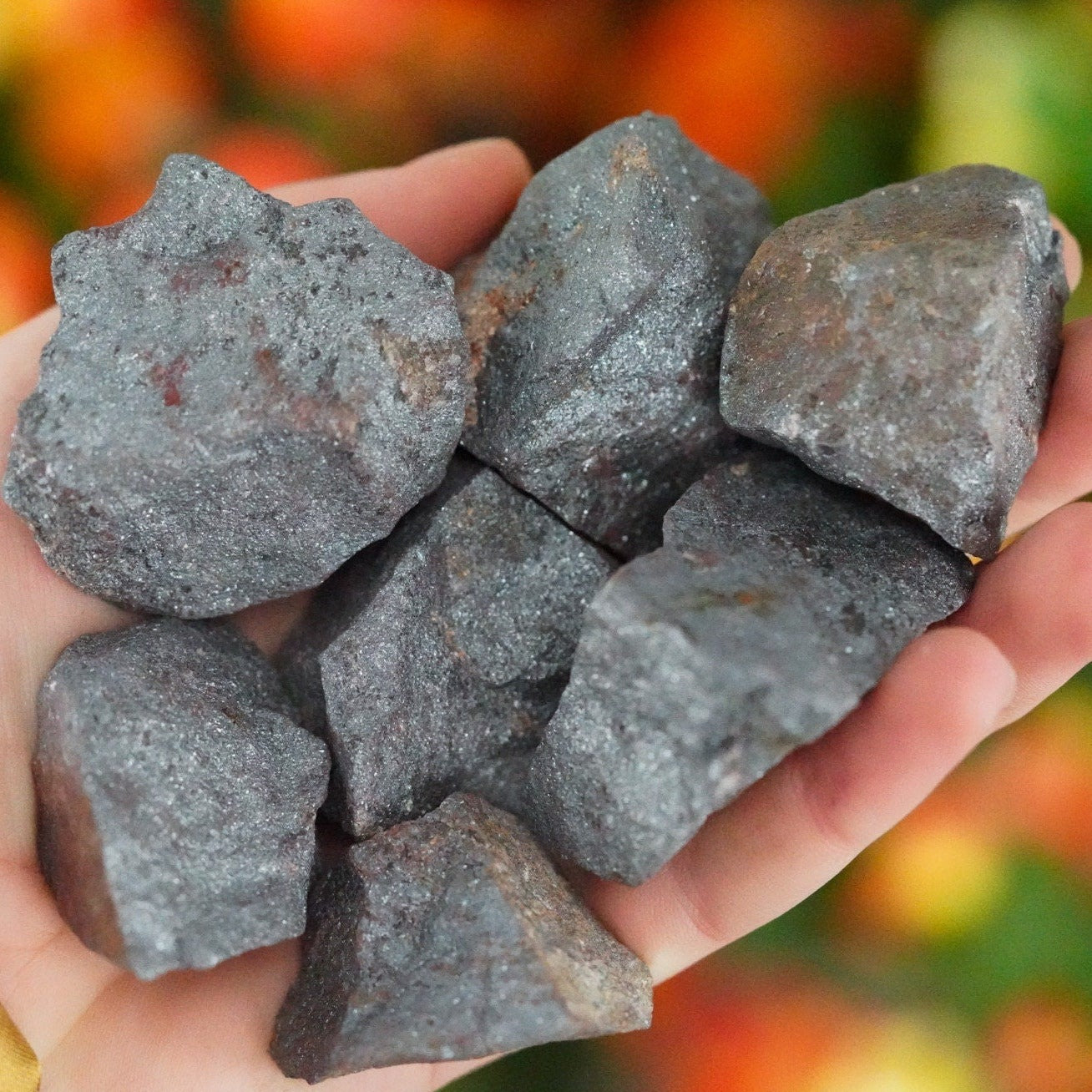A left hand, slightly cupped to prevent anything from falling, is holding seven large pieces of gravel—each roughly the size of a quarter or fifty-cent piece. These rocks are predominantly grey with some variations, including hints of brown, white, and red. The stones have shiny, silvery sheens and dark gray tones, with each one featuring a unique shape. The top rock also has distinct indent lines on it. The hand, filled with these granite-like stones, has its entire palm and fingers covered. The background of the image is blurred, with a striking red hue above the hand and patches of green and orange toward the bottom right.